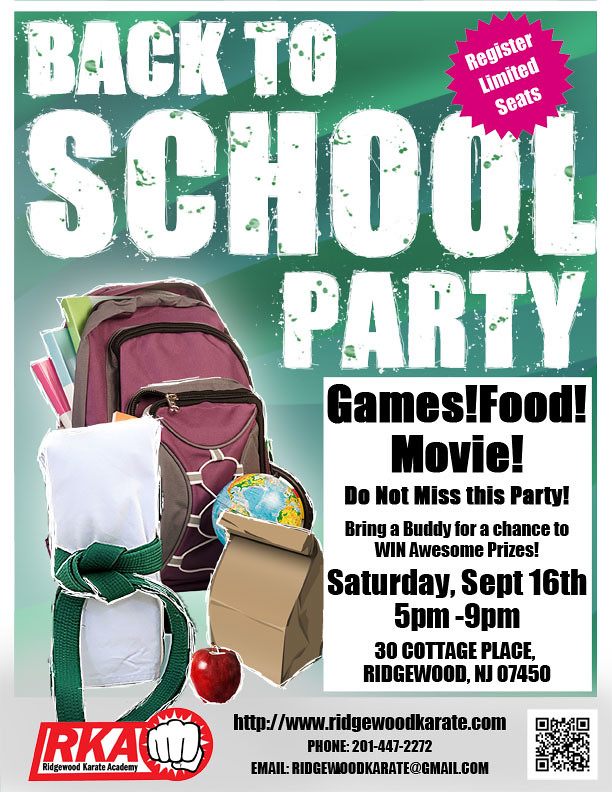This is a detailed flyer advertising a back-to-school party organized by RKA Ridgewood Karate Academy. The background transitions from light green and blue stripes at the top to gray at the bottom, setting a vibrant tone for the event. Bold, white text at the top announces, "Back to School Party," with a distinct scuffed look and a dark green dot pattern across the letters. The top right corner features a pink starburst design with angled white text stating, "Register Limited Seats."

On the left side, prominently featured, is an open purple backpack with green, blue, and pink packets visible, symbolizing back-to-school preparations. Alongside the backpack, there's a brown paper lunch bag folded over, a red apple, a globe in the background, and a white cloth bundle tied with a green ribbon, enhancing the visual appeal.

The right side of the flyer contains a white rectangular panel with black text listing the event's highlights: "Games! Food! Movie! Do not miss this party." The detailed schedule includes, "Saturday, September 16th, 5 PM to 9 PM," and the location, "30 Cottage Place, Ridgewood, New Jersey, 07450." Below this panel are contact details, including a barcode for easy access, the website www.ridgewoodkarate.com, phone number 201-447-2272, and email ridgewoodkarate@gmail.com.

The bottom left corner displays the red logo of RKA Ridgewood Karate Academy alongside a fist symbol, reinforcing the event's sponsor. The overall design effectively combines visual elements and essential information, creating an inviting and engaging advertisement for the upcoming party.